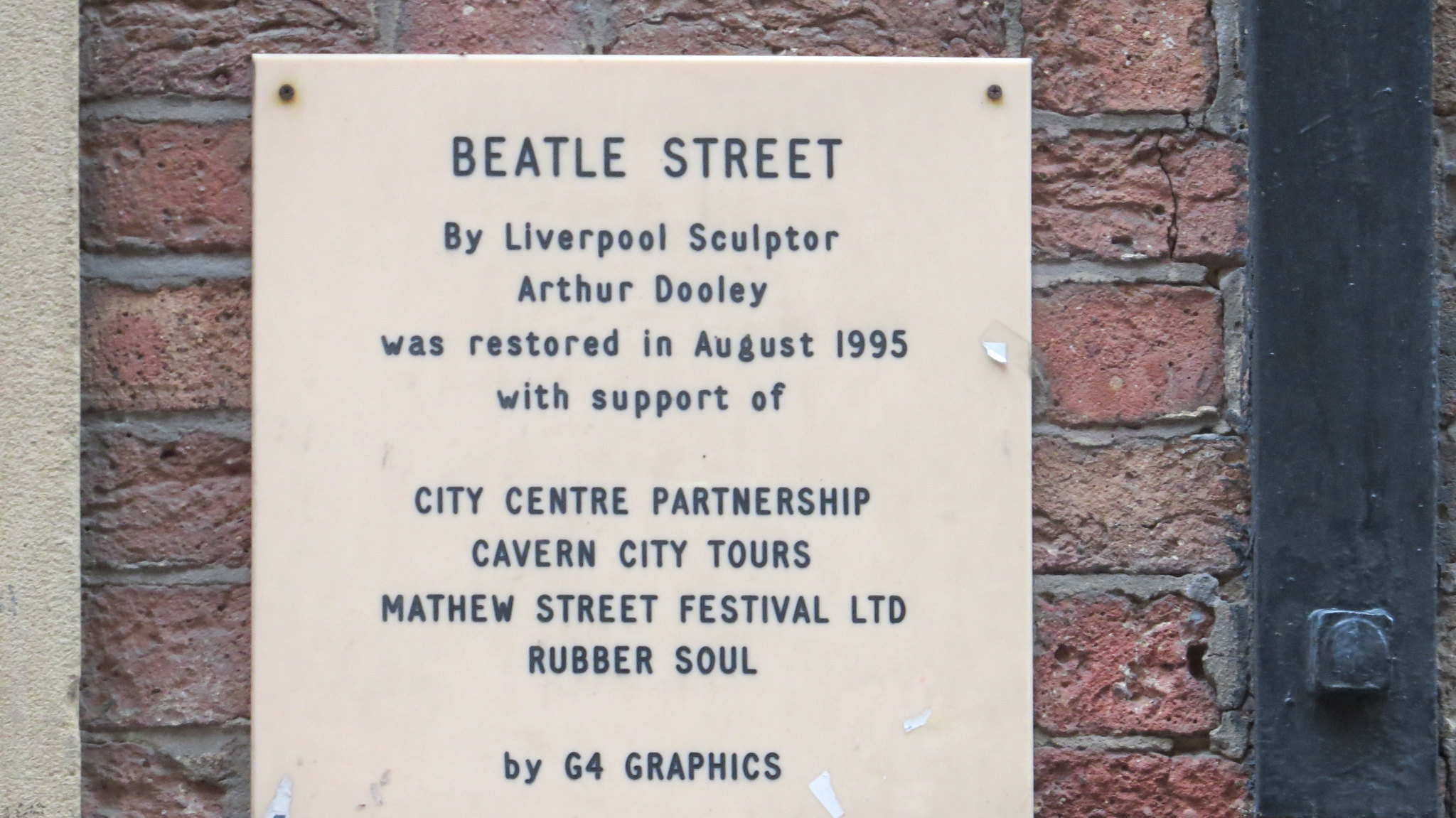This image shows a detailed brick wall with a prominently displayed white square plaque. The plaque, extensively inscribed in capital letters, reads: "Beatle Street by Liverpool sculptor Arthur Dooley was restored in August 1995 with the support of City Center Partnership, Cavern City Tours, Matthew Street Festival, LTD, Rubber Soul, by G4 Graphics." The clean white board it is mounted on contrasts sharply with the red bricks forming a backdrop. Off to the right, there are metal bars and what appears to be a very worn, black doorknob. The setting appears to be outdoors, likely on a street, as suggested by the plaque and surrounding architecture. The text on the plaque varies in boldness and coloration, predominantly featuring black letters. There are no people visible in the image, ensuring the focus remains on the sign and its historical significance.